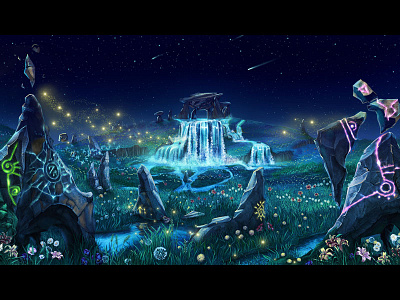The image portrays a captivating, fantasy landscape, meticulously crafted through digital art. At the heart of this enchanting scene, a luminous blue waterfall cascades into a stream that winds horizontally across the bottom, surrounded by grassy fields speckled with vibrant pink, yellow, and white flowers. Triangular rock formations, dark gray with enigmatic symbols illuminated in yellow and pink, frame the foreground. The night sky, painted in deep navy blue, is adorned with twinkling stars and the luminous trails of shooting comets. The ethereal atmosphere is heightened by the presence of glowing fireflies, adding a magical touch to this fairytale-like setting.